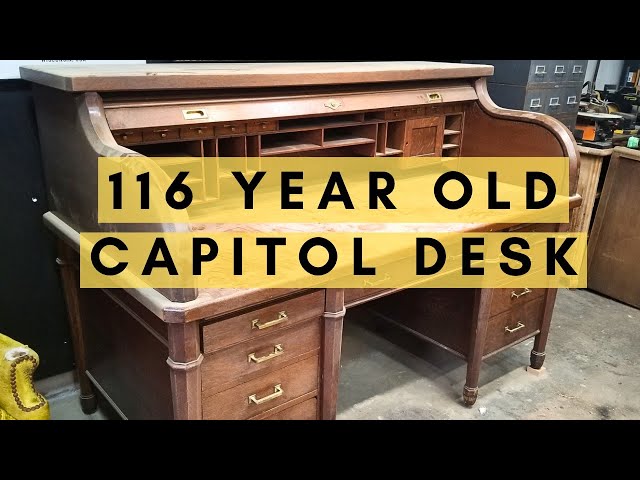The photograph captures an antique 116-year-old Capital Desk, prominently featured in an office setting. This roll-top desk, constructed entirely of wood, exhibits a rich brown hue complemented by gold handles. The distinctive roll-top is partially retracted, exposing a variety of small compartments ideal for sorting letters, cards, and office supplies, arranged in a neat, square pattern. The desk boasts multiple drawers, six on either side, flanking a central seating area, evoking the classic style of an old postman's workspace. Overlaying the image in yellow text with black lettering is a caption that reads "116-year-old Capital Desk," partially obscuring the detailed craftsmanship of the desk itself. The background reveals a concrete floor, gray metal filing cabinets, and what appears to be restoration equipment, indicating its current environment. Notably, to the left of the desk is a detail of a greenish-yellow leather chair. The setting suggests preparations for refinishing the desk, enhancing its potential as a treasured piece for an office or home.